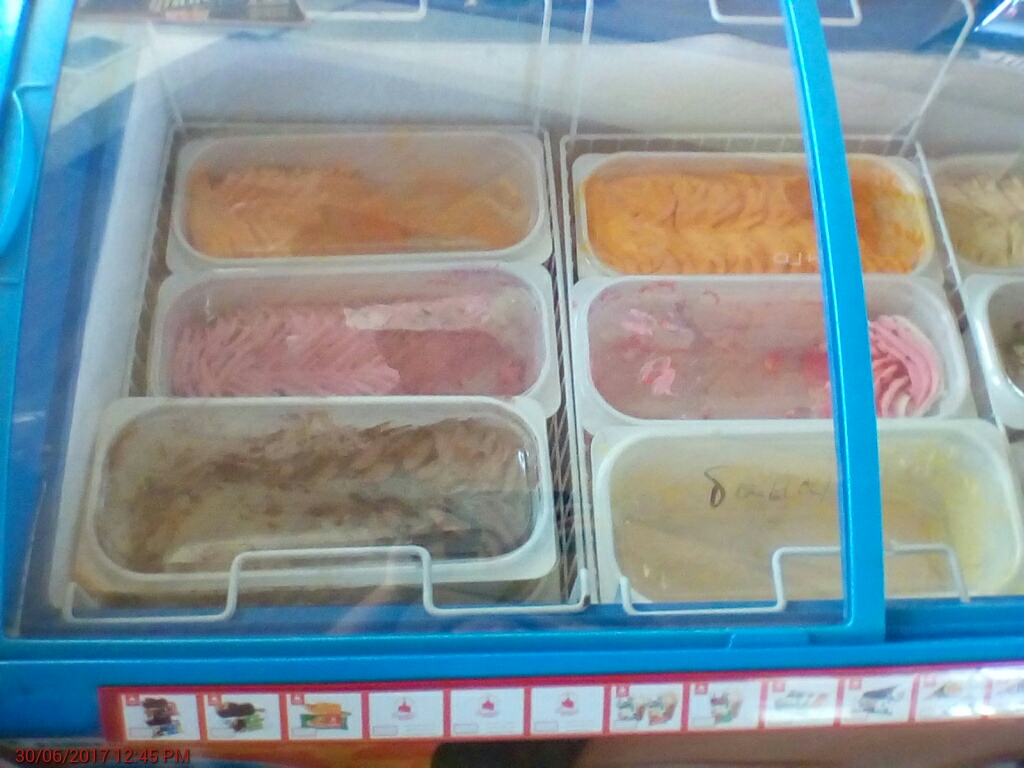This photograph showcases a store's ice cream cooler, composed of hard light blue plastic with a clear door that slides from left to right. Inside the cooler, six tubs of ice cream are prominently visible. The top two tubs contain orange ice cream, while the middle row features two tubs of strawberry ice cream. The bottom left tub appears to contain chocolate ice cream, with vanilla ice cream beside it on the right. Additional tubs are barely visible farther to the right, making it difficult to discern their flavors. At the very bottom of the freezer, there is a picture menu or a series of tags displaying the ice cream flavors or prices. The cooler is situated on what looks like a wooden floor.